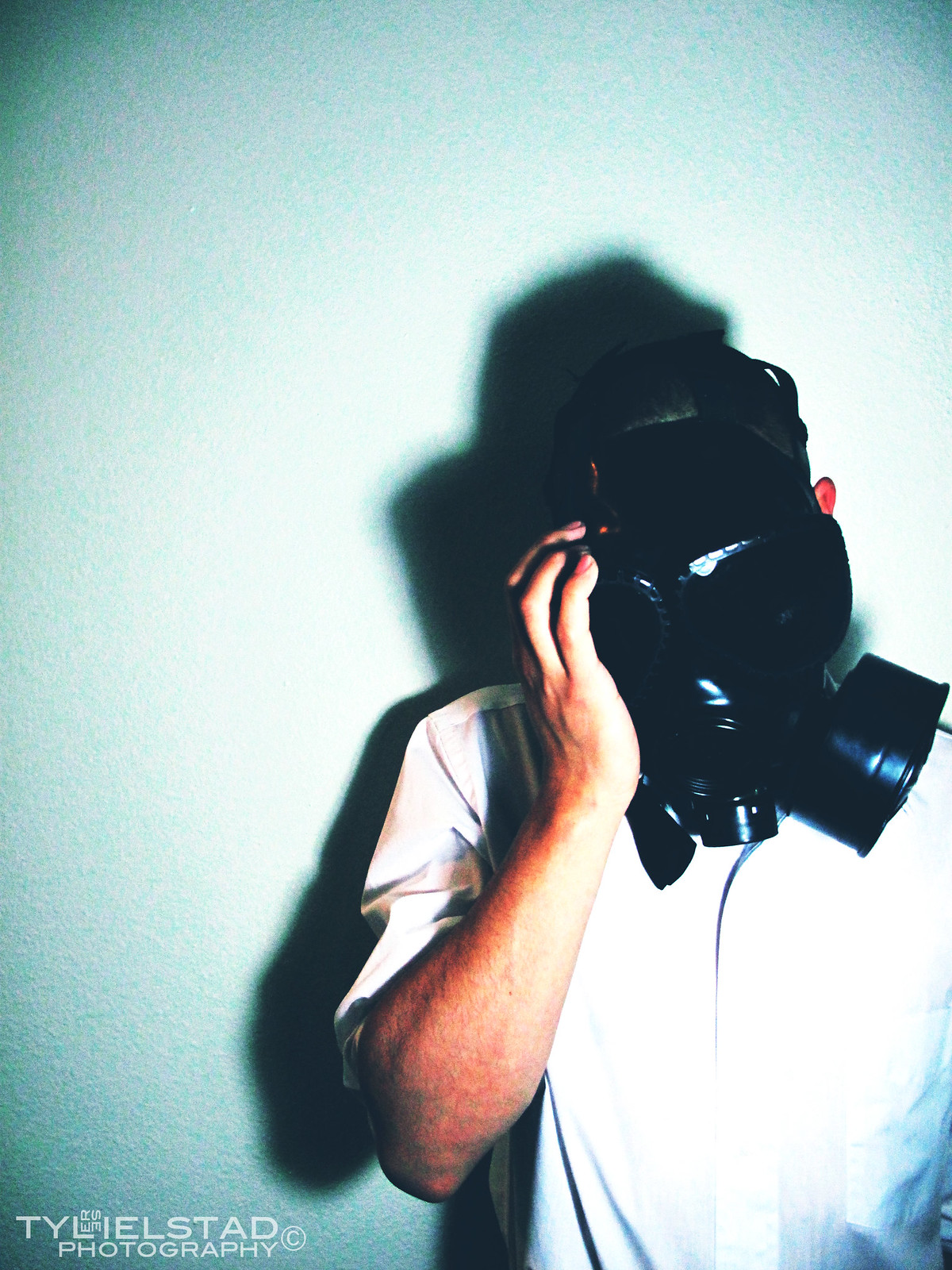In this color photograph taken indoors, a man is portrayed standing against a bluish wall or curtain that is lighter in the center. He has dark hair and is wearing a short-sleeved white shirt. His face is completely obscured by a black gas mask, the design of which covers his entire head. The man is holding his right hand up to the right side of the mask, near the eye holes but above the canisters, while the tip of his left ear is subtly visible. A spotlight casts a harsh shadow of both the man and the mask prominently behind him. At the bottom of the image, the text "Tylestad Photography" is visible, with a "C" in a circle indicating copyright.